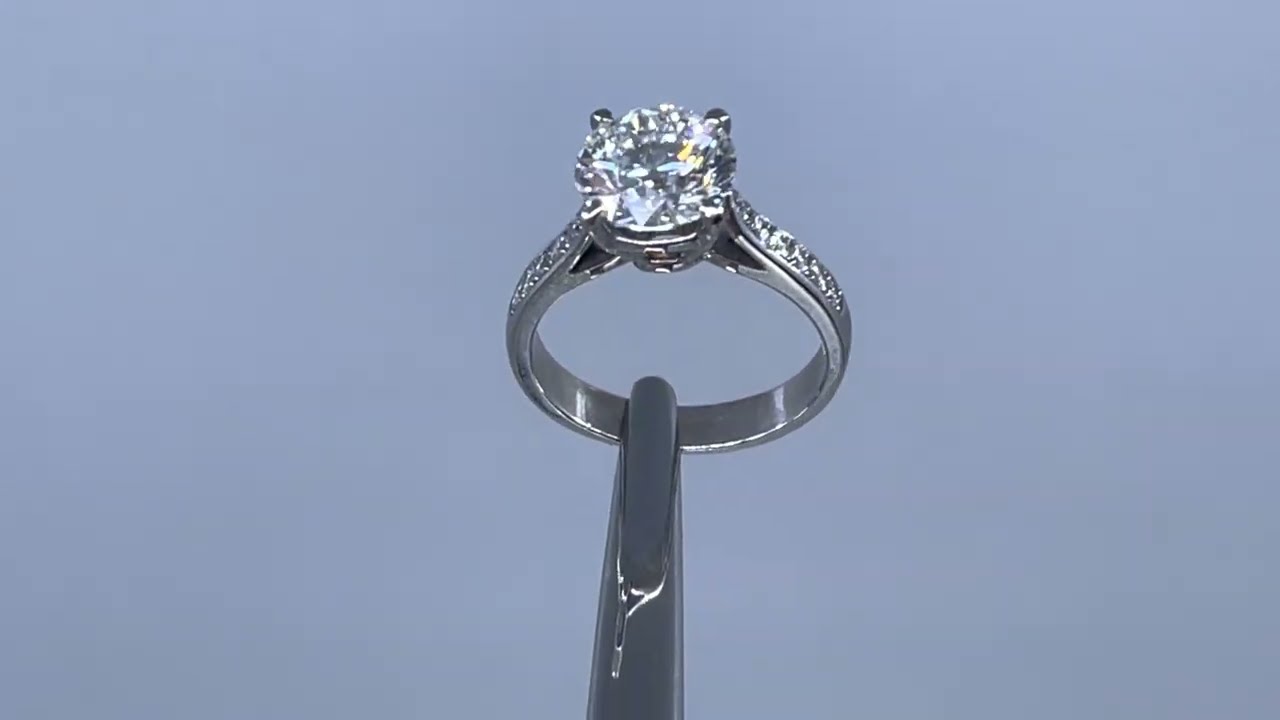In this close-up image, a stunning diamond engagement or wedding ring is showcased prominently against a light blue-gray background. The ring features a large, multifaceted diamond as its centerpiece, held securely in a four-prong setting that allows the sparkly gem to radiate an array of colors, including green, blue, white, and yellow. The band, likely made of platinum or a similar silver metal, is adorned with smaller diamonds set into the upper sides, adding to its overall brilliance and value. The ring is held delicately by silver tweezers, positioning it centrally within the frame. The image has a high-quality, polished appearance, suggesting it could be an advertisement or stock photo for a jewelry website.